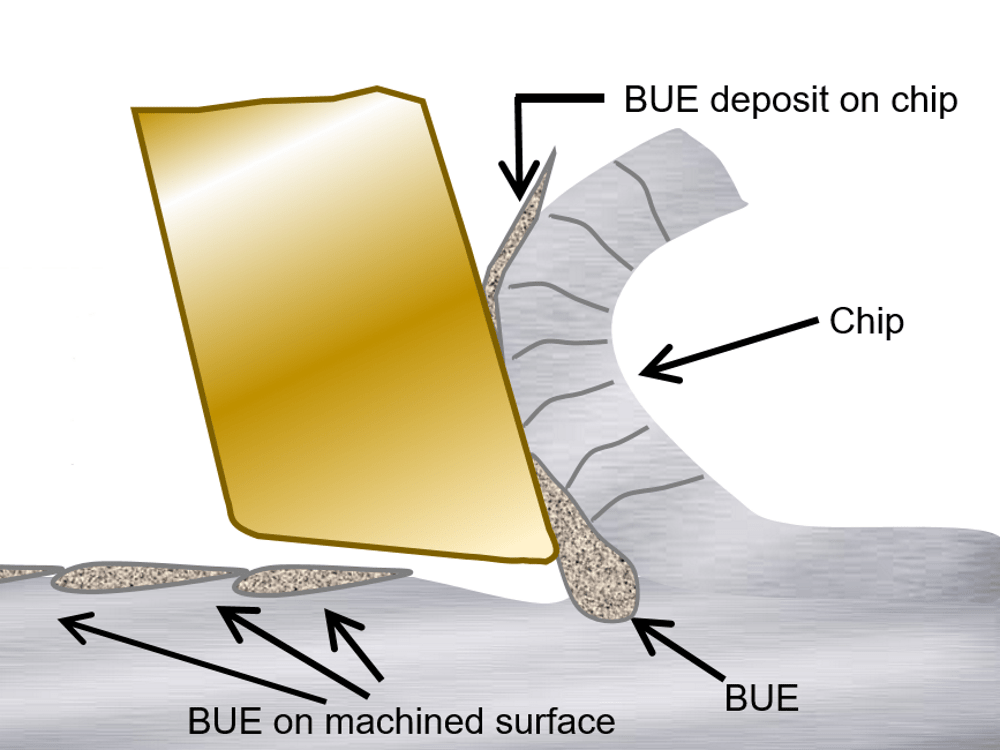The image features a detailed, labeled illustration highlighting various components and materials. At the center, there's a shiny gold piece shaped like a slanted rectangle with jagged edges, exhibiting shades of light gold, regular gold, and white, bordered by dark gold. On the right side of this gold piece, a curved gray structure, resembling a C-shaped cylinder, displays dark gray stripes running vertically. This gray part has small gray speckles scattered across it.

Several labels are present in the image. One label, "B U E deposit on chip," points to the area where the gray and gold parts intersect. Another label simply states "chip" and points to the striped gray structure. Additional labels, all reading "B U E," indicate the charcoal-speckled areas on the gray structure. On the left side of the image, the label "B U E on machined surface" is pointed towards by three arrows, directing attention to another part of the gray, speckled area. Overall, the image delineates the interaction between a machined gray surface and various deposits, primarily emphasizing the BUE (Built-Up Edge) phenomenon.